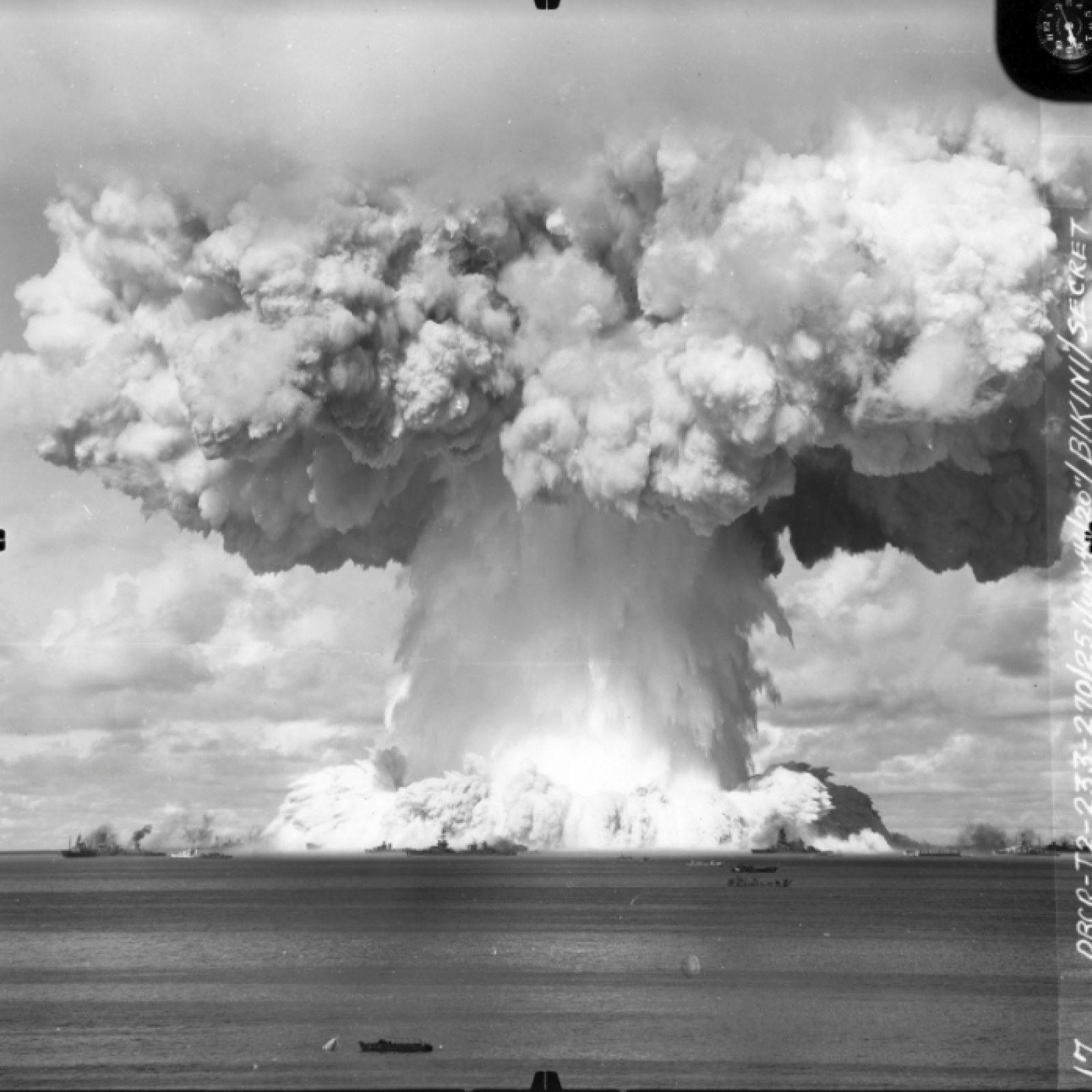This black and white photograph captures a monumental mushroom cloud resulting from an explosion on an island, obscuring the island almost entirely. The image foreground features water, likely part of an ocean, with boats scattered around the perimeter of the island. The focal point is the colossal mushroom cloud, with a thick stem rising centrally and billowing out into a vast, dense cap that dominates the sky. The cloud exhibits a range of shades from dark gray to pure white, blending with the cloudy sky. In the distant background, beyond the island, a shoreline with trees is faintly visible. Partially legible text on the side of the photograph reads, "17 [illegible letters/numbers] / bikini."